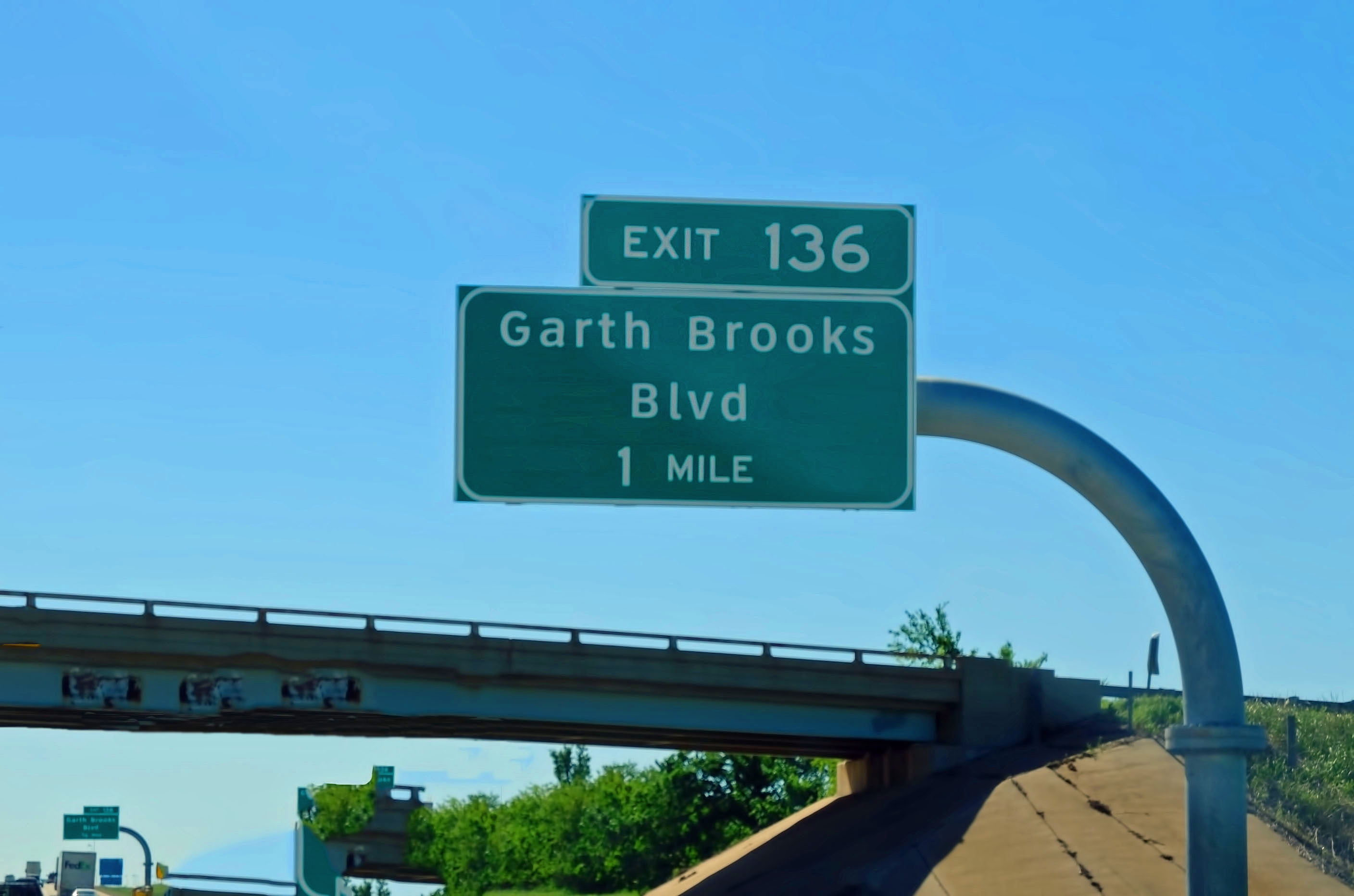This image captures a detailed, close-up view of a green highway sign perched on a silver, curved pole that extends upward and bends to the left, hanging over the highway. The main, rectangular sign is bordered in white and prominently displays "Garth Brooks Boulevard, one mile" in bold white text. Above this, a smaller rectangular sign reads "Exit 136." The scene also features a blue, cloudless sky that fades to a lighter turquoise near the horizon. Below the sign, an overpass spans the entire width of the image from left to right, casting a shadow on the concrete beneath it. The overpass is adorned with graffiti and surrounded by green vegetation. In the background, a long bridge stretches horizontally, flanked by clusters of trees. Distant highway signs, along with trucks and other vehicles, can be seen far off to the bottom left, while the sloping green grass on the right further enhances the sense of depth and distance in the photo.